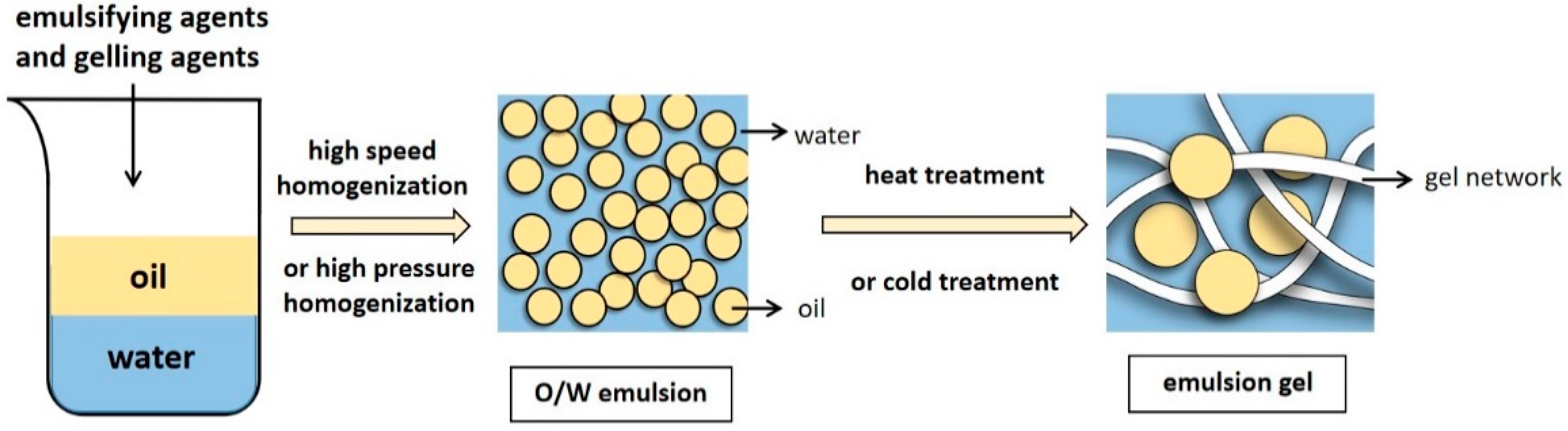This image clearly illustrates a three-step chemical process involving emulsification and gelling. The process begins with a depiction of a beaker, where water, shown in blue, and oil, depicted in yellow, are combined with emulsifying and gelling agents. An arrow labeled "high-speed homogenization" or "high-pressure homogenization" points to the next stage, where a mixture of small yellow oil droplets is suspended in blue water, forming an O/W (oil-in-water) emulsion. The final step involves either a heat or cold treatment, transforming the emulsion into an emulsion gel. In this stage, the oil droplets are interconnected by a network of white strands, indicative of the gel structure, with an arrow pointing to the term "gel network." This comprehensive visual representation details the transition from initial mixing through homogenization to the final gel formation.